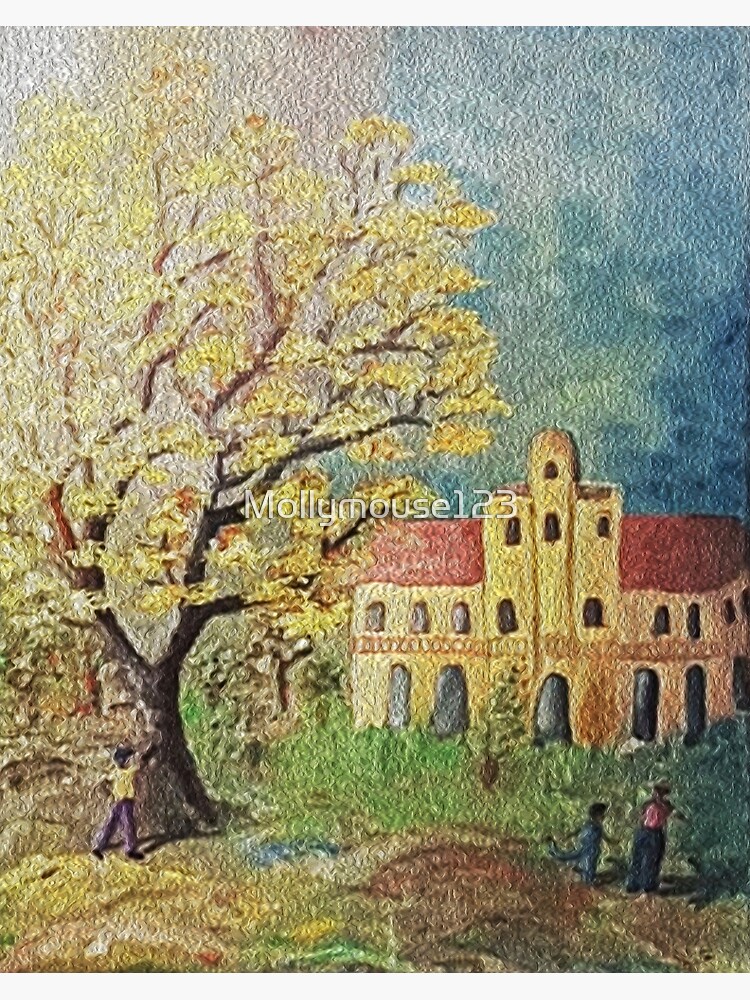This vertically oriented painting depicts a serene pastoral scene, prominently featuring a large tree with a brown-black trunk and yellow foliage positioned on the left side. To the right, a large villa or Spanish mission-style building is illustrated. This stone-based structure, with a distinctive red roof, has a three-story central section and an imposing four-story center tower, suggesting it might be a religious building. The facade of the building features a series of white arches on the first story and smaller, black windows on the upper stories, hinting at an interior courtyard.

In the foreground, two human figures stand on a mixed ground of yellow, brown, and blue hues. One figure with a yellow shirt and gray pants is positioned near the tree. To the right, another figure in a red shirt and blue pants stands alongside a smaller boy dressed in blue. Green foliage stretches across the area in front of the building, adding depth to the scene. Another smaller tree, marked by a black trunk and yellow leaves, is painted in front of the villa. The sky above is painted with a rich texture, transitioning from darker blue on the right to a beige hue on the left. The entire artwork holds a watermark in the middle, stating “Mollie Mouse 123.”